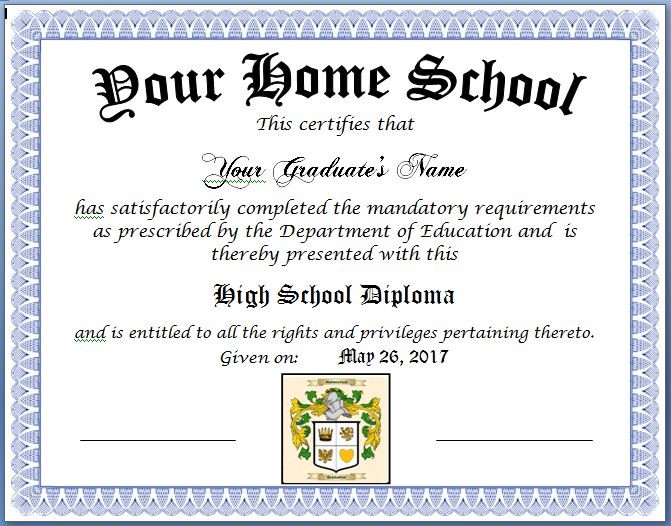The image showcases a high school diploma featuring a detailed design. At the top, the text reads "Your Home School." The diploma certifies that the graduate, referred to as "your graduate's name," has satisfactorily completed the mandatory requirements as prescribed by the Department of Education and is thus presented with this high school diploma, entitling them to all the rights and privileges that accompany it. This formal document is dated May 26, 2017.

Encircling the diploma is an ornate blue border, reminiscent of a certificate of appreciation. At the bottom center lies a crest, adorned with a green and yellow theme, featuring a knight’s helmet at its pinnacle. The crest is divided into four smaller sections, each containing an image, with a banner underneath that contains some text. Below the crest are two blank lines designated for signatures, likely reserved for school authorities. The overall appearance of the diploma includes a combination of black text in various fonts set against a white background.